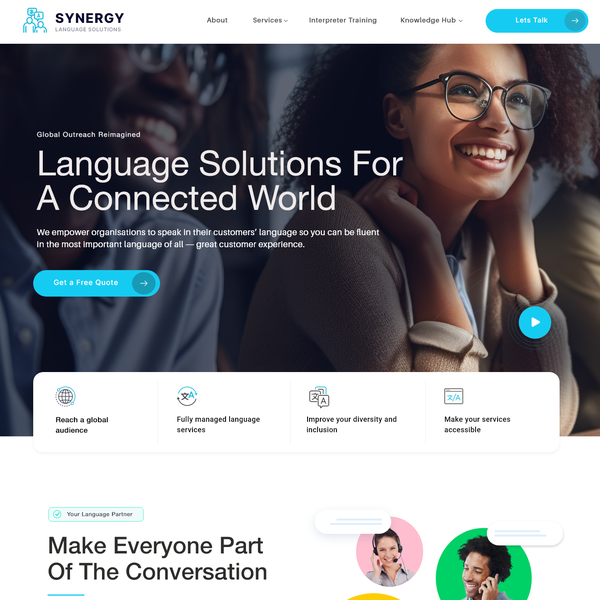This image from Synergy's website features a detailed layout designed for clarity and user engagement. The top inch of the image is bordered by a white strip. On the left, there are two small blue outlines of human figures, each above a numbered bubble—'3' for the first and '4' for the second.

To the right of these icons, "Synergy" is prominently displayed in bold, black letters, with the tagline "language solutions" in smaller, black type below it. Approximately an inch to the right, the menu options "About," "Services," "Interpreter Training," and "Knowledge Hub" are listed in small black font. A blue tab labeled "Let's Talk" with a right-pointing arrow in white is also present.

Below this header, there is an image featuring two individuals. On the left is an African-American man, smiling broadly and wearing glasses, a blue shirt, and a black tie. To his right is a woman with shoulder-length hair, also smiling, wearing glasses and a long-sleeved brown shirt, with her hands up to her cheeks. On one of her wrists is a blue circle with a white play button icon. Across the man’s smile, the text "global outreach reimagined" is written in small white letters.

Below this, large white text reads "Language solutions for a connected world." Further down, two lines of information are displayed in small white font, accompanied by a blue tab that says "Get a free quote" in white letters.

At the bottom of the picture, a white rectangle extends across the width, featuring four icons and their corresponding labels. Directly beneath this, the background turns entirely white. On the left side, the text "Make everyone part of the conversation" is visible. Adjacent to this text, there are two profile pictures: one of a girl with a headset on a pink background and another of an African-American man holding a phone to his ear, smiling, against a green background.